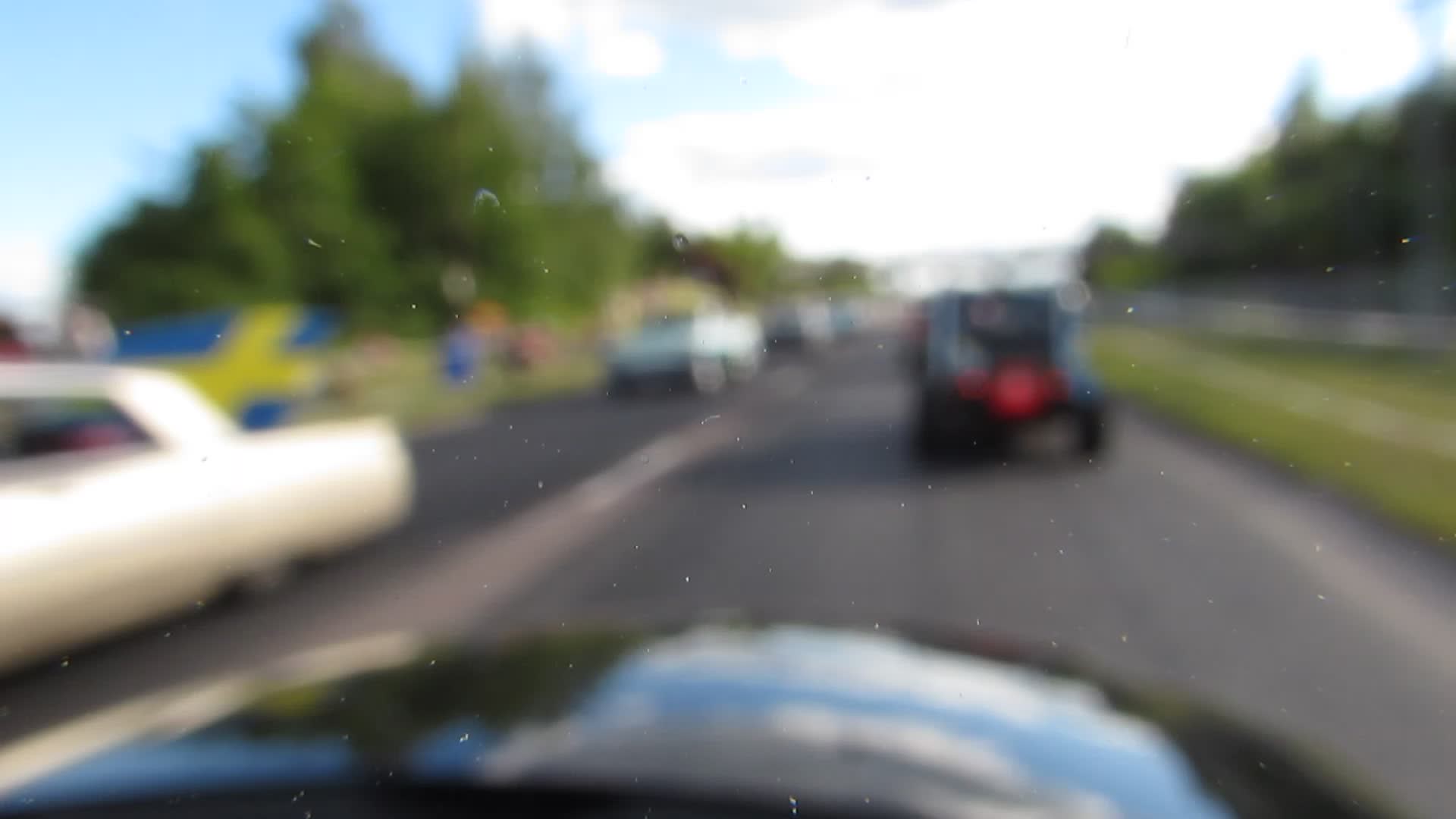This blurry photograph, captured through the front windshield of a moving vehicle, shows a scene on a two-way highway flanked by trees. To the left, a 1960s era sedan with a long trunk and distinctive wheel covers is visible, traveling towards the camera. This white classic car is followed by another vehicle, possibly light blue, but indistinct due to the blurriness. Straight ahead on the pavement, a car with its brake lights on is seen, indicating slow movement in traffic. The scene is set against a backdrop of greenery with grass and large trees lining both sides of the road, extending into the distance. Above, the sky is a bright blue with scattered white clouds, adding contrast to the otherwise muted, blurry traffic scene.